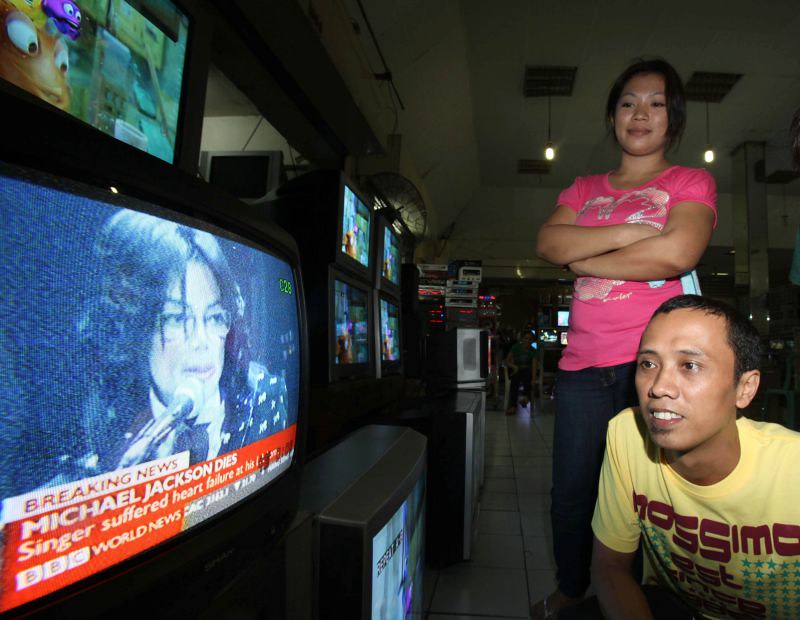In a brightly lit electronic store, a man and a woman are engrossed in a television screen displaying breaking news. The screen, situated on the left side of the room, shows a black-and-white video of Michael Jackson with a red banner below stating "Breaking News: Michael Jackson died. Singer suffered heart failure at..." followed by "BBC World News." The woman, standing behind the man, is dressed in a pink shirt and black pants. She has dark black hair that covers her ears and a warm smile on her face, her arms crossed over her stomach. The man, positioned in the lower right corner, is wearing a yellow t-shirt adorned with dark amber-colored letters and green stars. Surrounding them are multiple other televisions, some displaying colorful images of purple and brown animals with big blue eyes. In the background, two yellow lights hang from the ceiling, adding a warm glow to the scene. Various computer equipment is stacked up in the rear of the room, and the floor is made up of white tiles with grey grout in between.